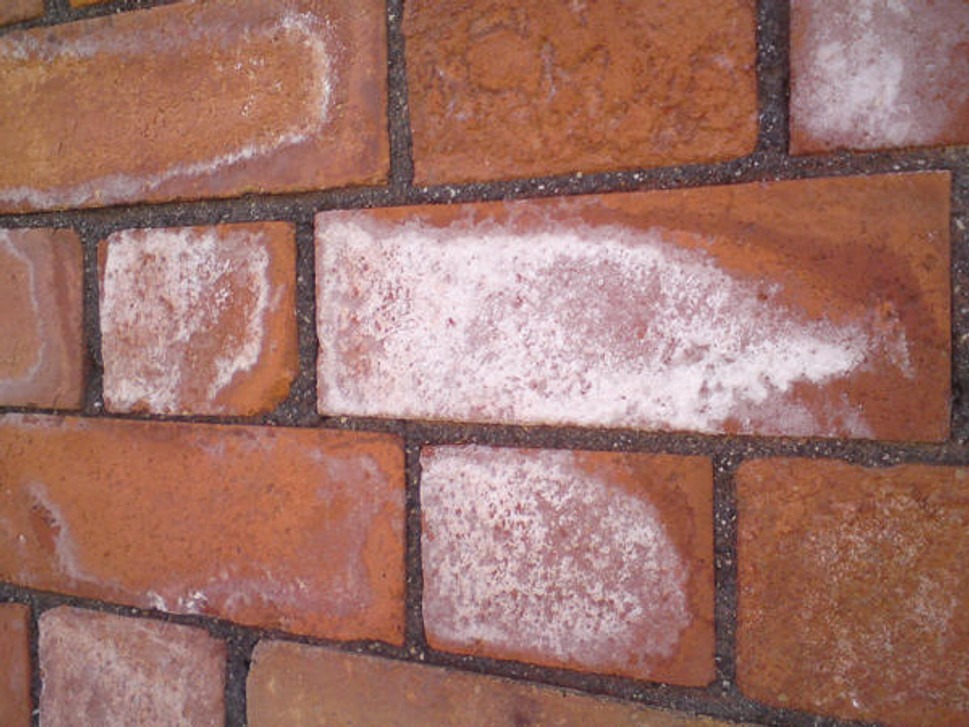The photograph showcases a detailed view of a cemented brick wall primarily composed of dark red bricks of varying sizes. The majority of the bricks are rectangular, interspersed with a few smaller, square-shaped ones. The bricks are held together with a dark brown or grayish cement that adds a granular texture to the wall's surface. An area of the wall features white stains, which could be indicative of mold growth or residual paint. The wall also appears to be slightly damp, suggesting recent drying. The overall setting reflects a construction or building style.